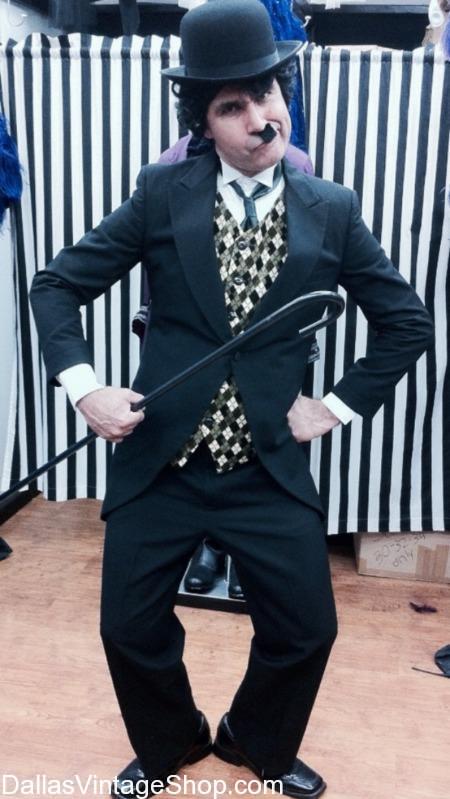The photograph features a Charlie Chaplin impersonator striking the iconic pose. The man has a distinctive appearance reminiscent of Chaplin, with a small mustache just below his nose and a playful, exaggerated facial expression. He is dressed in a black suit comprising black dress pants, a black jacket, a checkered vest over a white dress shirt, and a blue tie. Adding to his Chaplin look, he dons a rounded black top hat and holds a black cane in his right hand. His legs are bent slightly, and his feet form a V shape, with his hands placed firmly on his hips. His hair is curly and black, aligning with the vintage style he's emulating. The background includes a black-and-white striped curtain, with the bottom edge revealing another pair of black shoes. The floor is wooden, adding to the vintage feel of the scene. In the bottom left corner of the image, white text reads "dallasvintageshop.com."